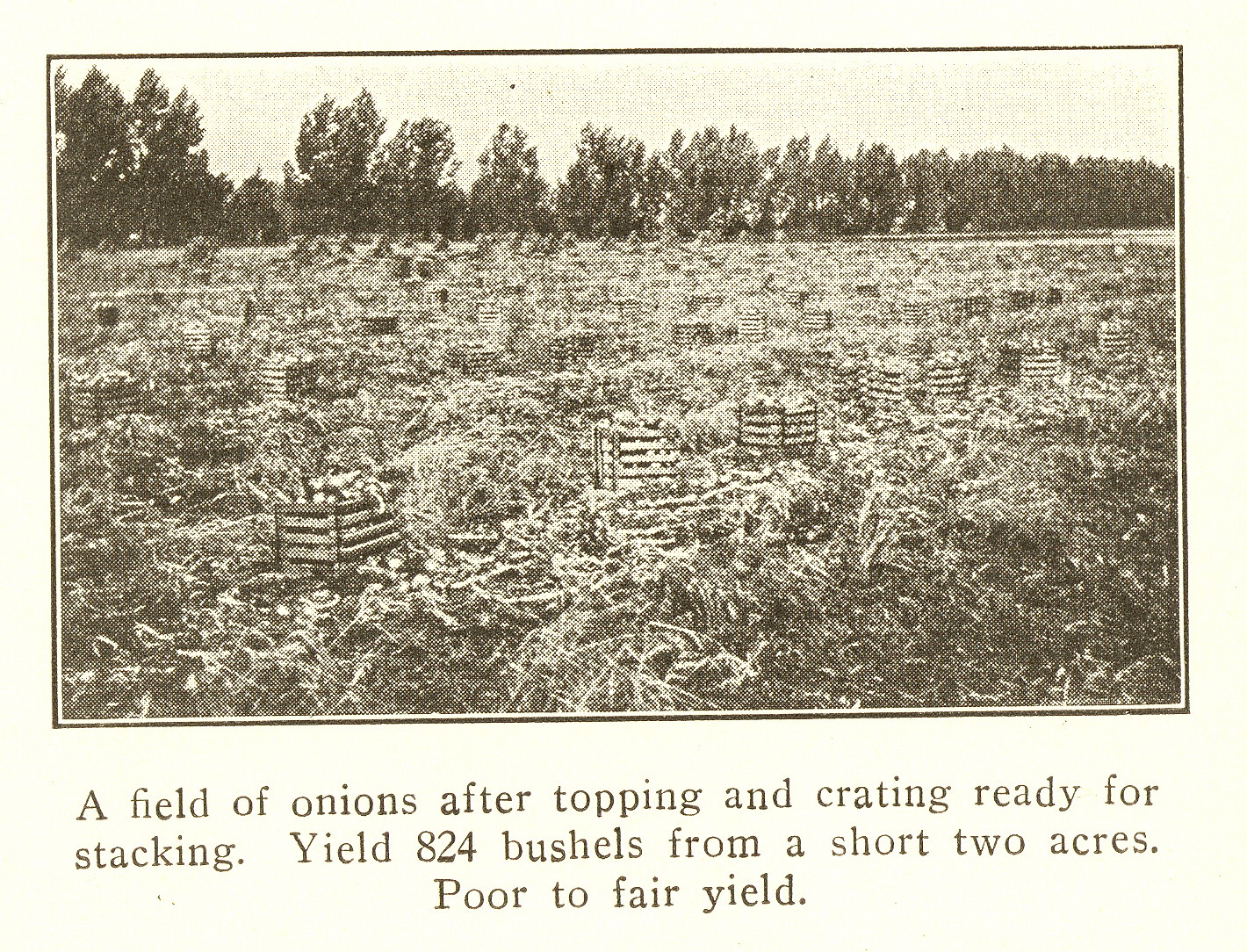This image appears to be a sepia-toned, black-and-white photograph depicting an onion field, which seems like a scan of an old book or magazine page, given the pixelation and pale yellow background. The field, positioned centrally in the image, is scattered with various wooden structures, likely crates, and topped onions, indicating a yield of 824 bushels from a short two acres, described as poor to fair. The backdrop features a tree line and an expansive sky above. The photograph is dated and has a somewhat washed-out appearance, with black and white text at the bottom providing the caption: "A yield of onions after topping and crating, ready for stacking. Yield 824 bushels from a short two acres. Poor to fair yield." The framing is marked by a black rectangular border, and a notable black speck is present just left of the center near the top. The overall composition suggests the onion field fades into the distance, with individual elements becoming less discernible.